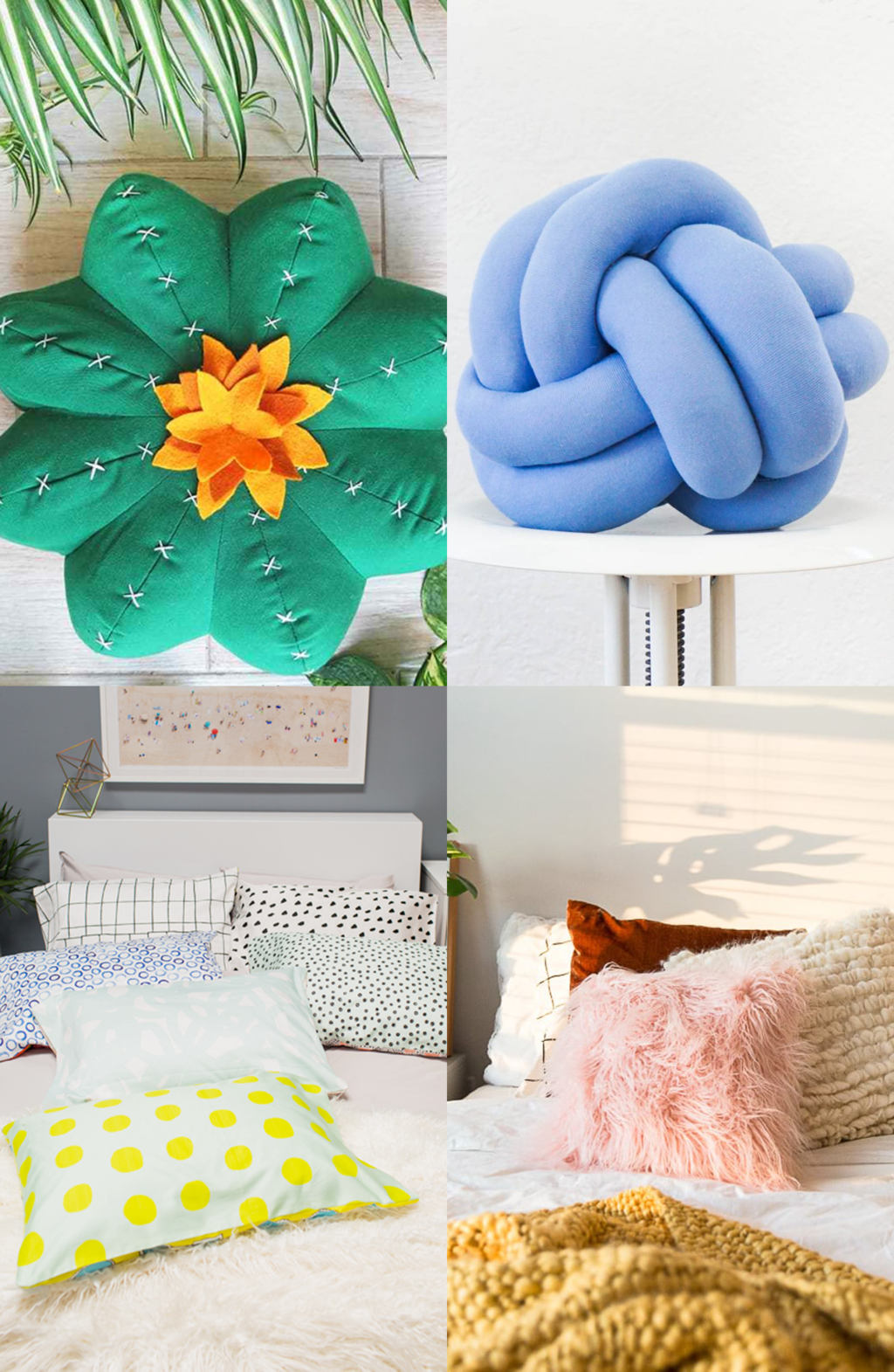The image is a composite of four vertically-aligned photographs depicting various pillows and bedding setups, arranged in a 2x2 grid. In the upper left quadrant, there is a star-shaped, green pillow featuring white X-shaped stitches along the seams of its eight petals. The center showcases three layers of felt-like flower shapes in varying shades of orange, with some green leaves in the background. Adjacent to it, in the upper right quadrant, is a unique, knotted pillow made of thick, blue, noodle-like tubes intricately wrapped together, resting on a white, round table.

The bottom half of the composite contains images of two different beds adorned with an array of decorative pillows. The bottom left image shows a bed cluttered with a variety of patterned pillows, including green and white plaid, white with large green dots, white with shades of blue circles, white with smaller green dots, and green with white shapes. Additionally, there's a white pillow with yellow polka dots and a fur blanket draped across the bed. The bottom right image features a more haphazardly made bed with fewer but distinct pillows: a white and gold plaid, a reddish-brown knitted pillow, a white pillow, and a unique pink shaggy pillow, all complemented by a yellow knitted blanket casually spread on the bed.